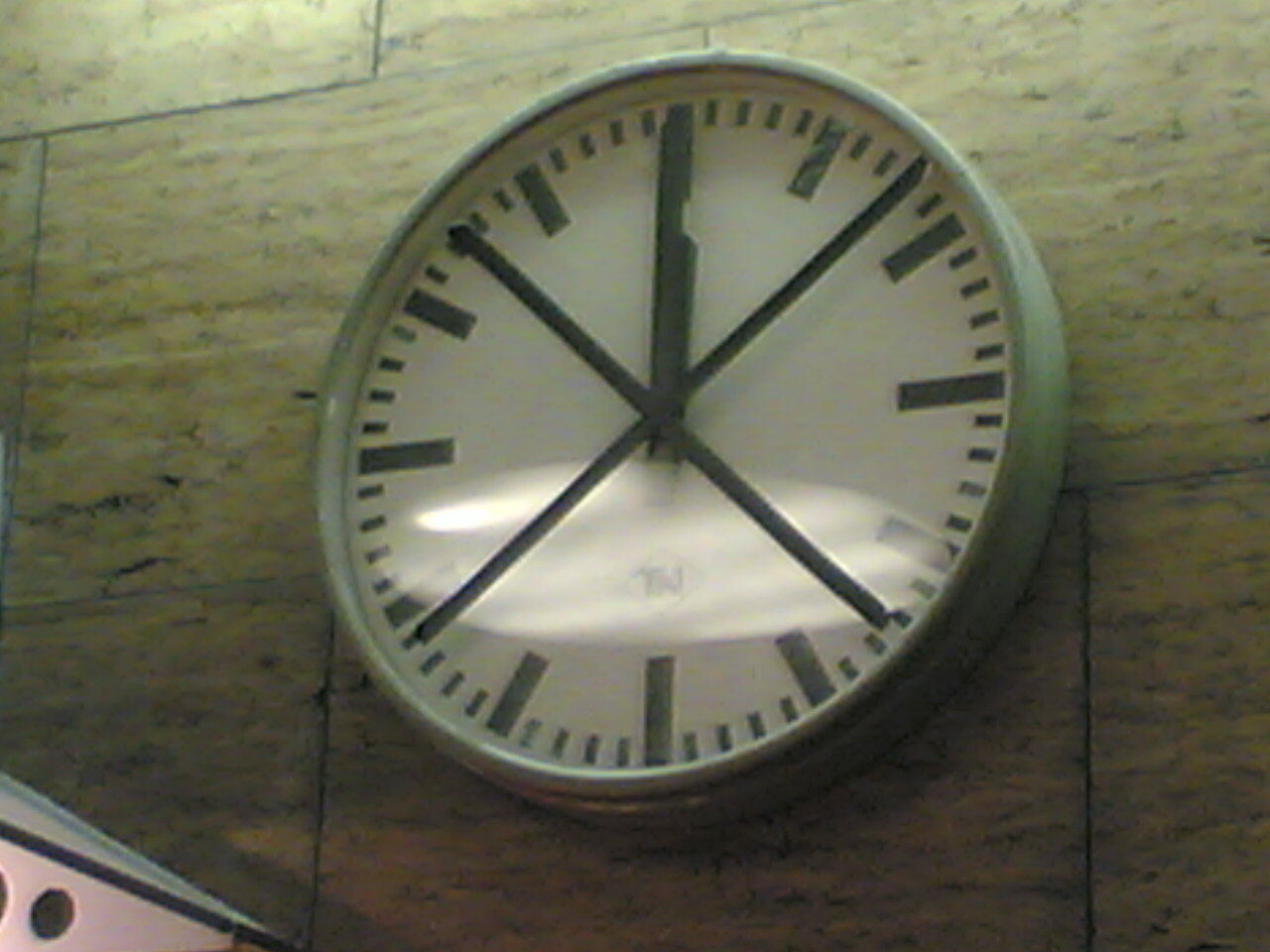This image depicts a close-up view of a round clock mounted on a wall composed of stone blocks, which exhibit a distinct stone pattern. The clock's casing appears to be made of plastic and is grayish in color. Marking the hours, the clock features thick lines in place of traditional numerals. A prominent black X intersects the center of the clock face. Both the hour and minute hands point precisely to 12 o'clock, suggesting that the time is noon or midnight. A subtle reflection of a light source within the room can be seen on the lower part of the clock face.